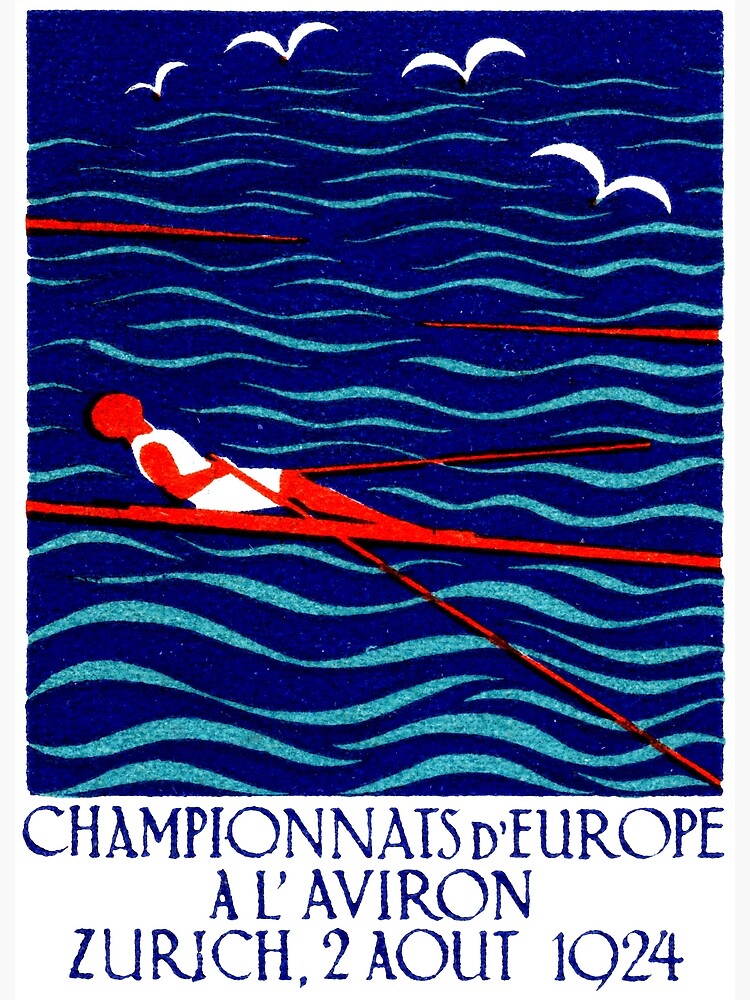This image appears to be a vintage poster from a 1924 European rowing championship in Zurich, titled "Championnat d'Europe de l'Aviron, Zurich, 2.08.1924." The design features a vivid blend of dark blue and light blue shades, representing the water with horizontal, wavy lines indicating movement. At the top of the composition, four white seagulls are depicted flying across a lighter blue sky. Central to the artwork is a red and white figure of a rower, illustrated with elongated, red oars. The figure's position and the oars suggest they are rowing backwards, propelling a boat across the water. Additional visual elements include a couple of red lines running through the blue waves, adding dynamic tension to the scene. The lower third of the poster contains the aforementioned text, framing the upper two-thirds, which dominantly feature the artistic depiction of the rowing event.